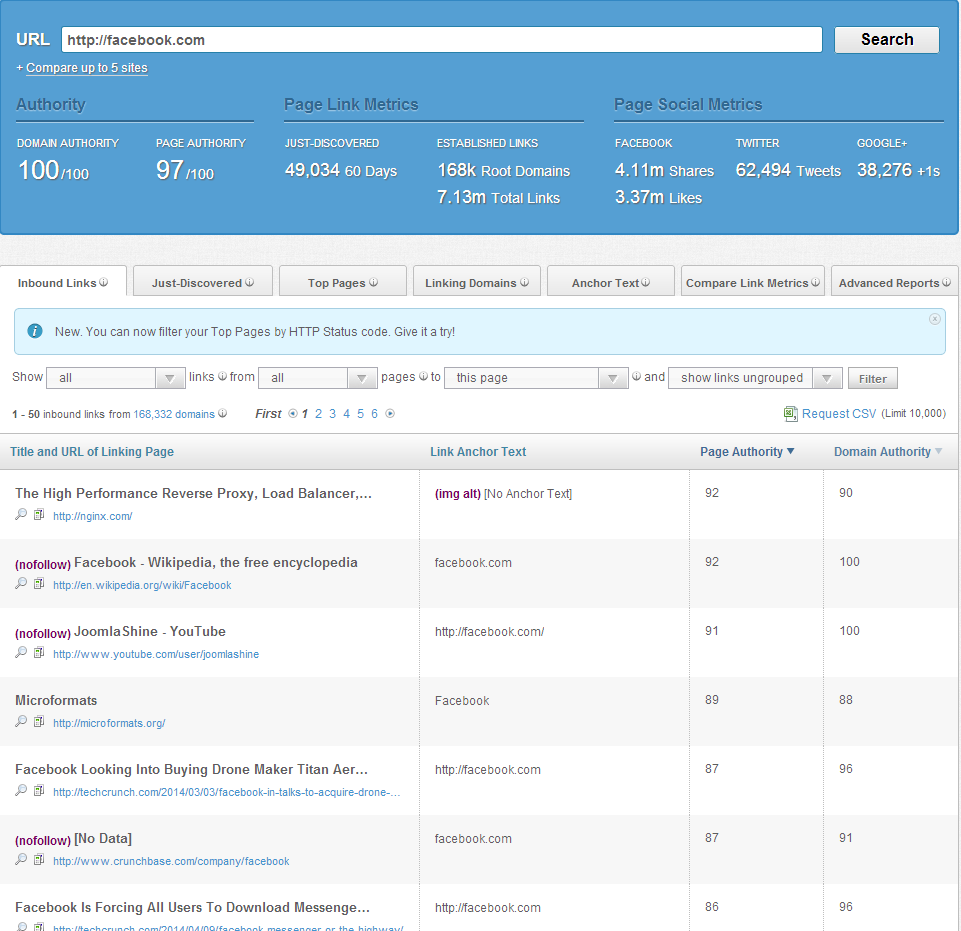The screenshot displays a website analytic tool. The top left corner shows "URL" in white text, set against a sky-blue background. A search bar prominently displays "facebook.com" with a grey "search" button on the far right. Below the search bar, there are three sections labeled: "Authority," "Page Link Metrics," and "Page Social Metrics."

In the "Authority" section, "Domain Authority" is rated 100 out of 100, and "Page Authority" is rated 97 out of 100. The "Page Link Metrics" section reveals two categories: "Just Discovered" links, totaling 49,034 in the past 60 days, and "Established Links," which includes 168,000 root domains and 7.13 million total links.

The "Page Social Metrics" section tracks social media interactions across three platforms:
1. Facebook: 4.11 million shares and 3.37 million likes.
2. Twitter: 62,494 tweets.
3. Google Plus: 38,276 +1s.

Below these metrics, there are various tabs featuring titles such as "URL," "Link Ranking Page," "Link Anchor Text," "Page Authority," and "Domain Authority," providing detailed information about the links and their respective metrics.